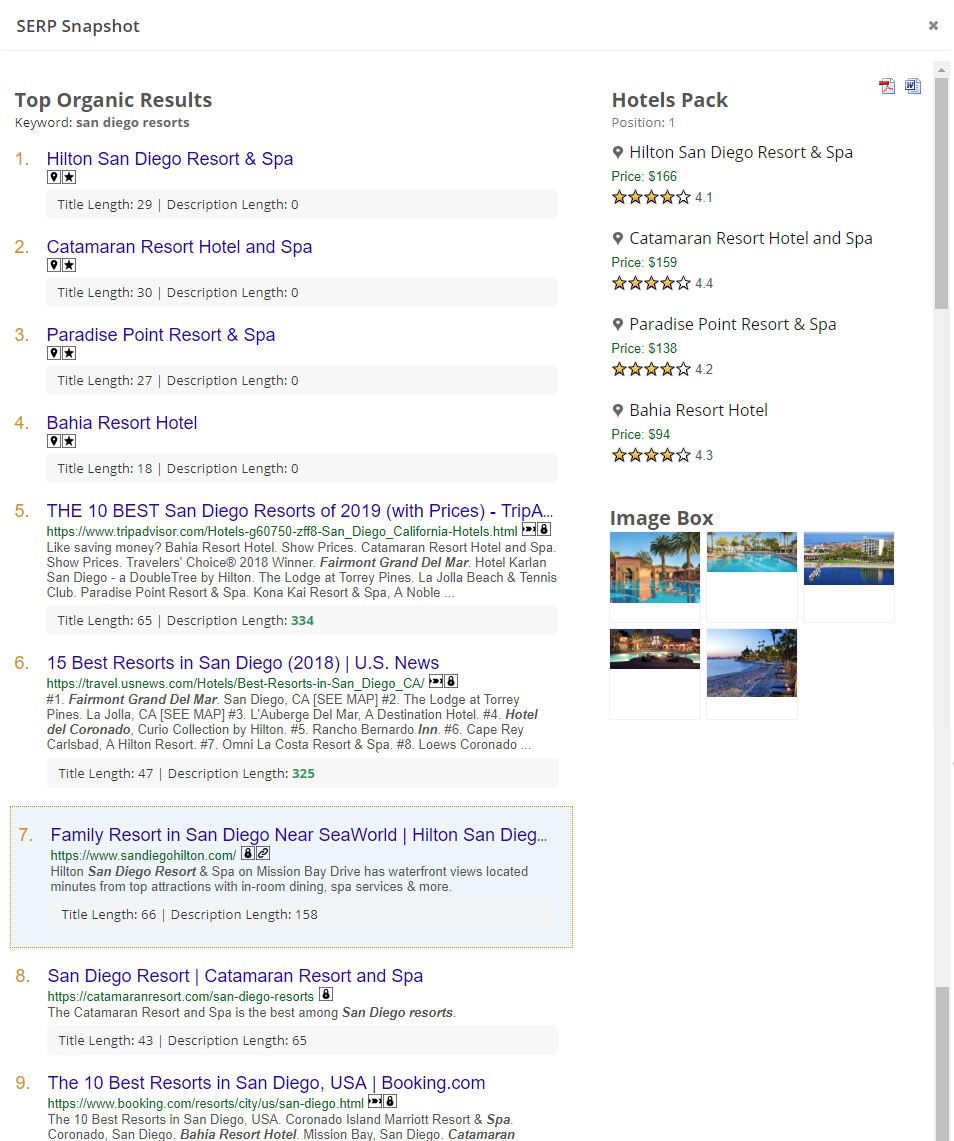The image showcases a webpage displaying search results from a browser. The page features a clean, solid white background. At the upper left corner, gray text reads "SERP Snapshot." Directly beneath, bold dark gray text states "Top Organic Results," followed by smaller gray text indicating the keyword "San Diego Resorts" in bold.

Beneath this heading, there is a list of nine results, each featuring a header in dark blue. The links are:
1. Hilton San Diego Resort and Spa
2. Catamaran Resort, Hotel, and Spa
3. Paradise Point Resort and Spa
4. Bahia Resort Hotel
5. The 10 Best San Diego Resorts of 2019 [with Prices]
6. 15 Best Resorts in San Diego [2018] (U.S. News)
7. Family Resort in San Diego near SeaWorld, Hilton San Diego
8. San Diego Resort, Catamaran Resort, and Spa
9. The 10 Best Resorts in San Diego, USA (Booking.com)

To the right of this list is another section labeled "Hotels Pack" in bold dark gray text. Below this heading, smaller gray text indicates "Position 1." This section lists several hotels with black text for names and green text for pricing, accompanied by star ratings represented in bright gold for filled stars. The hotels listed are:
1. Hilton San Diego Resort and Spa - $166 - 4 stars
2. Catamaran Resort, Hotel, and Spa - $159 - 4 stars
3. Paradise Point Resort and Spa - $138 - 4 stars
4. Bahia Resort Hotel - $94 - 4 stars

Further down, bold dark gray text reads "Image Box," under which several colorful images of various resorts are displayed.